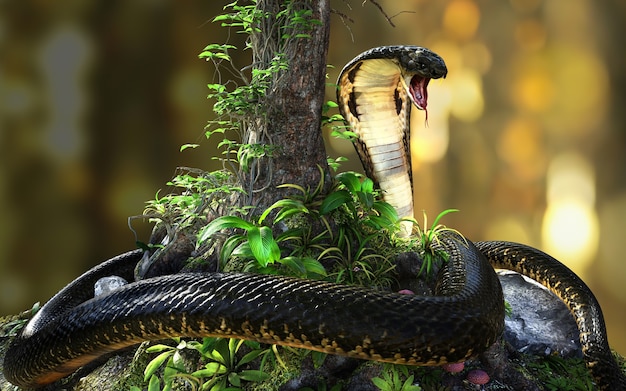In the center of this photograph, a striking black cobra is prominently featured as it curls around the slim trunk of a small tree. The snake's glistening black body contrasts sharply with its lighter yellowish-white underside, which is marked with sporadic black accents where it meets the snake's flared neck frill. The cobra's head is raised, its mouth wide open in a hiss, showcasing its fangs and protruding tongue. The detailed scales are clearly visible, emphasizing the snake’s menacing presence. Around the tree’s base and interspersed along its trunk, vibrant green leafy weeds add a touch of natural complexity. On the right side of the image, the snake’s tail extends and curves around a gray rock. The background is artistically blurred, featuring indistinct hues of gray, brown, yellow, and orange, with soft balls of light, creating a complementary yet unobtrusive backdrop.